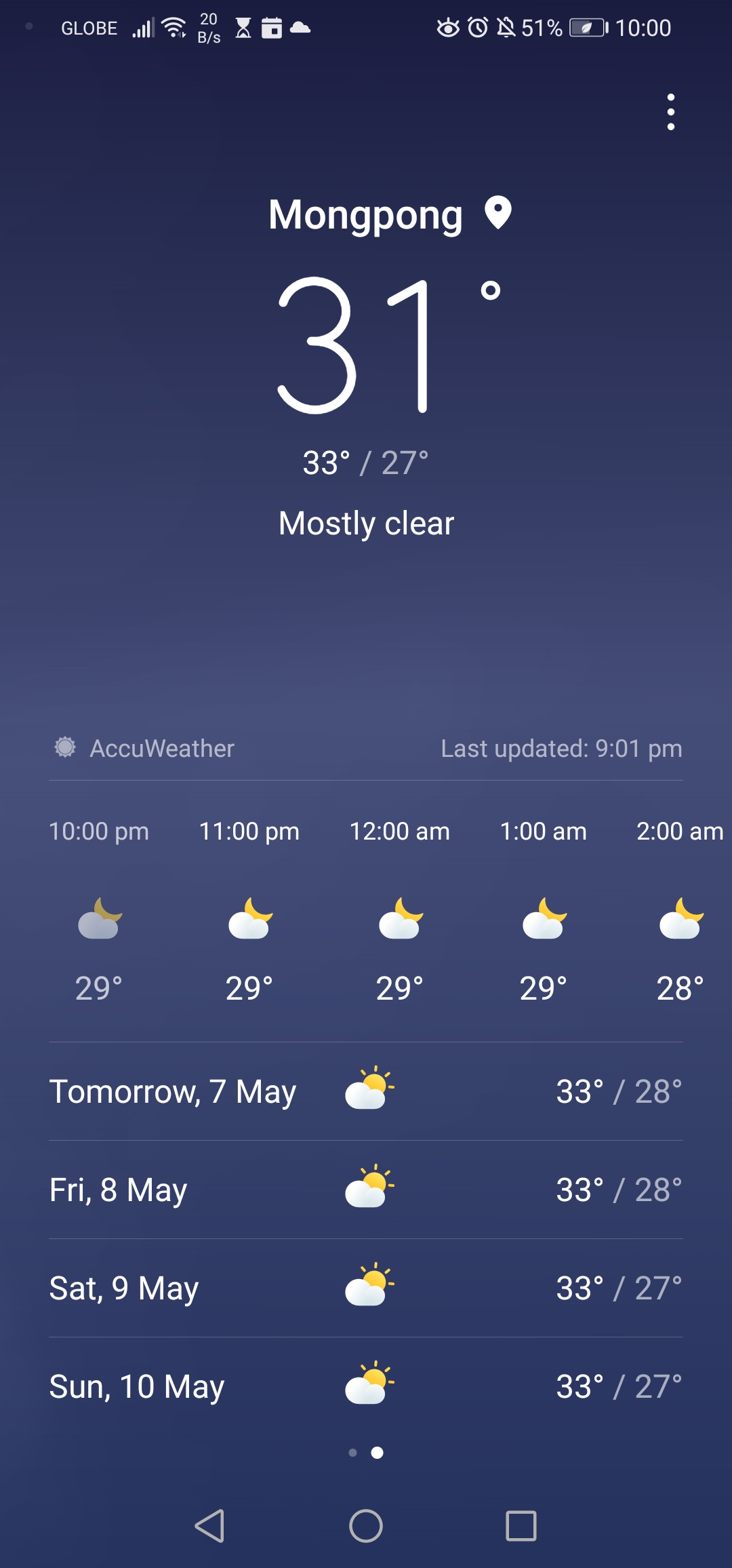The image displays a mobile weather app interface against a dark blue background. Starting from the top left, there's the text "Globe" in white. To the right, there are cellular signal bars, a Wi-Fi symbol, the number “20” with “B/S” below it, an hourglass icon, a file icon, and a cloud illustration. 

On the top right of the screen, there’s an eye icon, an alarm clock, a bell with a slash through it, the text "51%," a battery indicator with a leaf drawing inside it, and the time "10:00". Just below that, there's a vertical arrangement of three dots.

In the center, "Mong Pong" is displayed with a location marker icon next to it. Below this, the temperature is indicated as "31°C", and the min/max temperature is "33°/27°". The weather condition is described as "Mostly Clear".

The bottom section features the text "AccuWeather" on the left and "Last updated 9:01PM" on the right. Further down, there are hourly listings for different times (10PM, 11PM, 12AM, 1AM, 2AM) with corresponding temperatures. Additionally, there are daily listings with temperatures for upcoming days: tomorrow (7 May), Friday (8 May), Saturday (9 May), and Sunday (10 May).